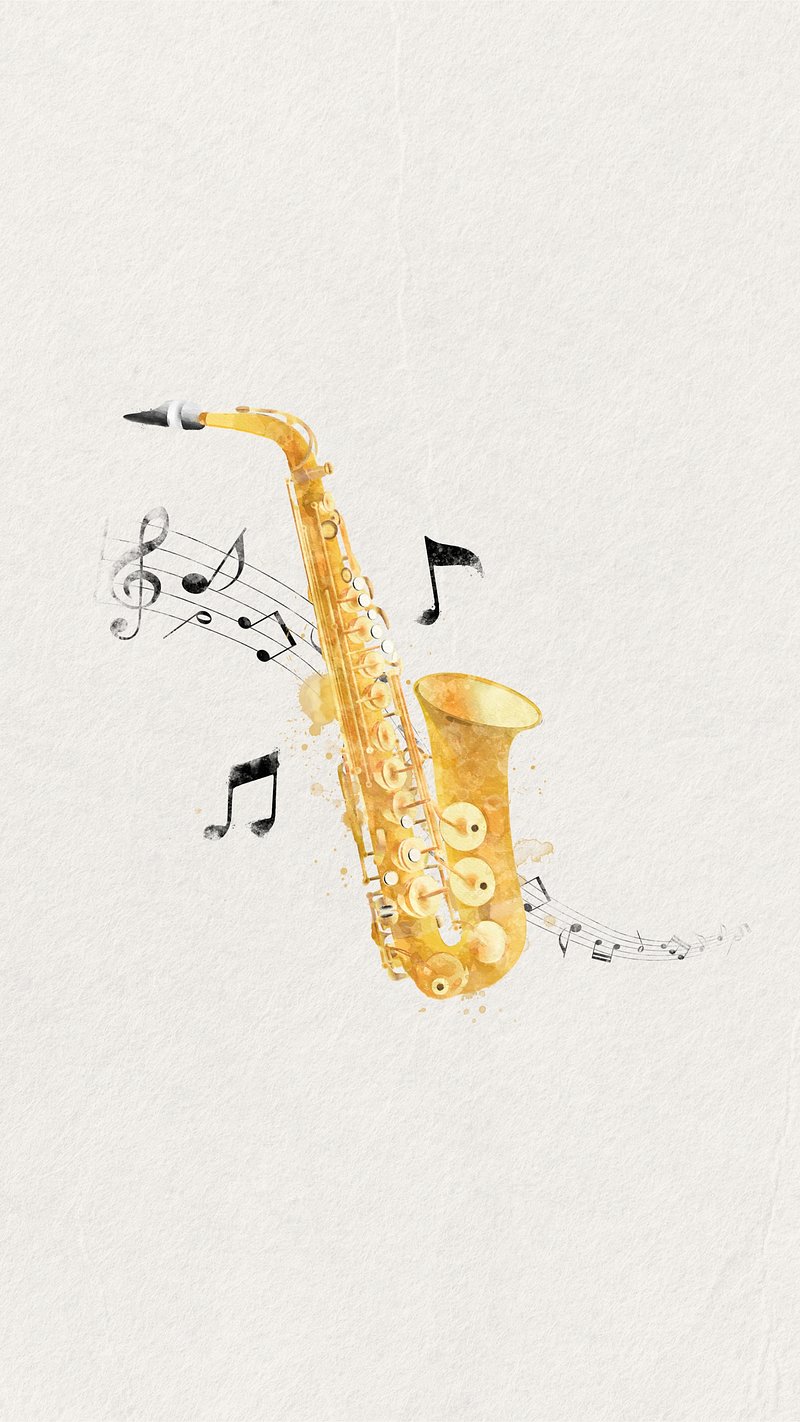This image features an exquisitely detailed drawing or painting of a golden-yellow saxophone, prominently centered against a plain white background. The saxophone's mouthpiece is a stark, dark black, and intricate lines and shading enhance its realistic appearance. Surrounding the saxophone, music notes appear to dance on a music staff, primarily starting from the upper left corner and elegantly descending to the bottom right. Apart from these, two additional music notes float freely, adding to the dynamic sense of musicality. The notes, including eighth notes and double notes, suggest an ongoing melody. A treble clef is noticeable towards the left side of the notes, further emphasizing the musical theme. The background remains void of any text, ensuring all focus remains on the central saxophone and its harmonious surroundings.